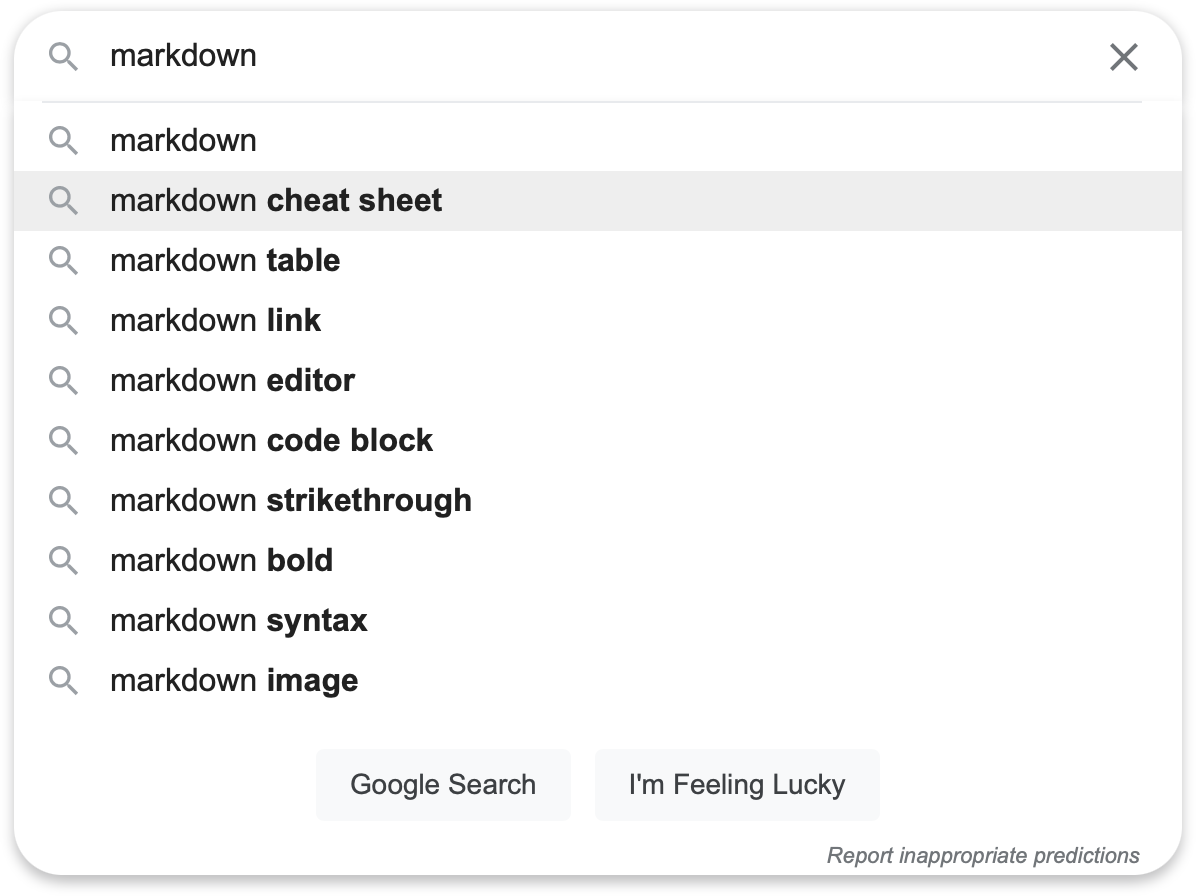The image depicts a Google search results page. At the top, spanning from the left to right, is the search bar. On the far left of the search bar is a light gray magnifying glass icon, and on the far right is a light gray 'X' button. The search query "Markdown" is displayed in black text within the search bar.

Below the search bar, there are several search results listed vertically. The results include "Markdown," "Markdown Cheat Sheet," "Markdown Table," "Markdown Link," "Markdown Editor," "Markdown Code Block," "Markdown Strike Through," "Markdown Bold," "Markdown Syntax," and "Markdown Image." The currently selected result, "Markdown Cheat Sheet," is highlighted with a grayish background that stretches horizontally across the width of the search results area. Each result is accompanied by a light gray magnifying glass icon to its left.

At the bottom center of the image, there are two rectangular buttons: "Google Search" on the left and "I'm Feeling Lucky" on the right. In the bottom right corner of the image, there is a light gray text that reads "Report Inappropriate Predictions."